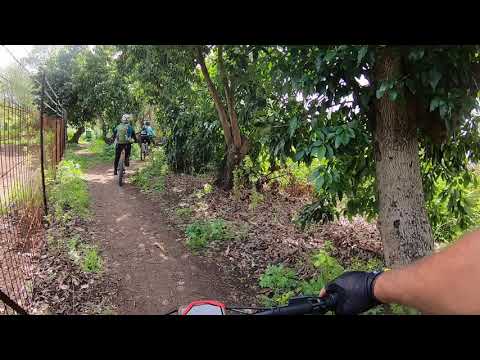This image captures a daytime scene from the perspective of a cyclist riding along a narrow, brown dirt path. The right hand of the cyclist, clad in a black glove, grips the black handlebars of a bicycle with a black frame. To the left of the path stands a weathered, metal fence topped with barbed wire, suggesting private property. To the right, a line of trees and scattered shrubbery frame the trail, their leaves creating patches of sunlight filtering through from above. The path, seemingly winding forward and then veering to the right, is populated by three to five fellow cyclists wearing helmets and jackets. The ground beneath their tires is dotted with weeds and fallen leaves, adding to the rustic, natural ambiance of the scene.